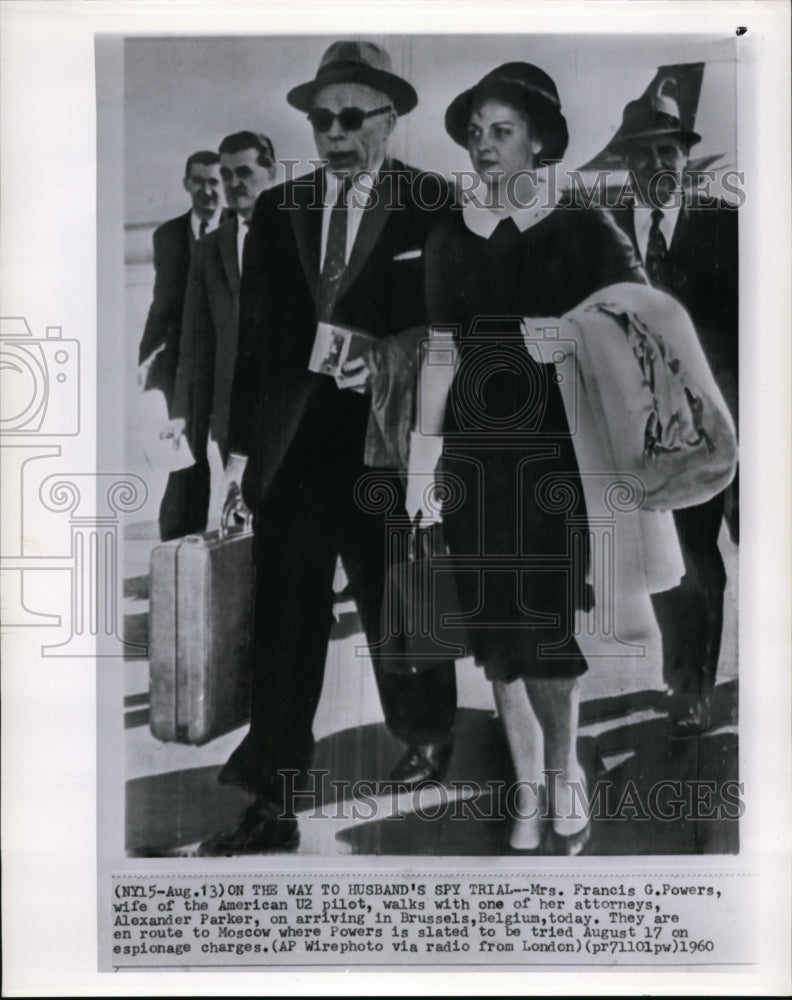This black-and-white vintage photograph, appearing as a newspaper clipping from August 13, 1960, captures a moment of historical significance. The image shows Mrs. Frances G. Powers, the wife of American U-2 pilot Gary Powers, walking alongside one of her attorneys, Alexander Parker. They have just arrived in Brussels, Belgium and are en route to Moscow, where Gary Powers is scheduled to face an espionage trial on August 17th. Mrs. Powers, a middle-aged Caucasian woman dressed in a knee-length black dress with a white lace collar, white gloves, a brimmed pillbox hat, and large pearl earrings, carries a handbag in her right hand and a fur coat draped over her left arm. Beside her is Alexander Parker, an older Caucasian gentleman in his 50s, wearing a dark suit, a white button-down shirt with a narrow dark tie, a fedora hat, and sunglasses. He holds a suitcase in his right hand and what appears to be airplane tickets in his left. Behind them, smaller in the background, are three similarly dressed men and the tail section of an airplane. The caption underneath the photograph details the context: "On the way to husband's spy trial, Mrs. Frances G. Powers, wife of the American pilot, walks with one of her attorneys, Alexander Parker, on arriving in Brussels, Belgium today. They are en route to Moscow where Powers is slated to be tried August 17 on espionage charges. (AP wire photo via radio from London) (PR7110PW)."